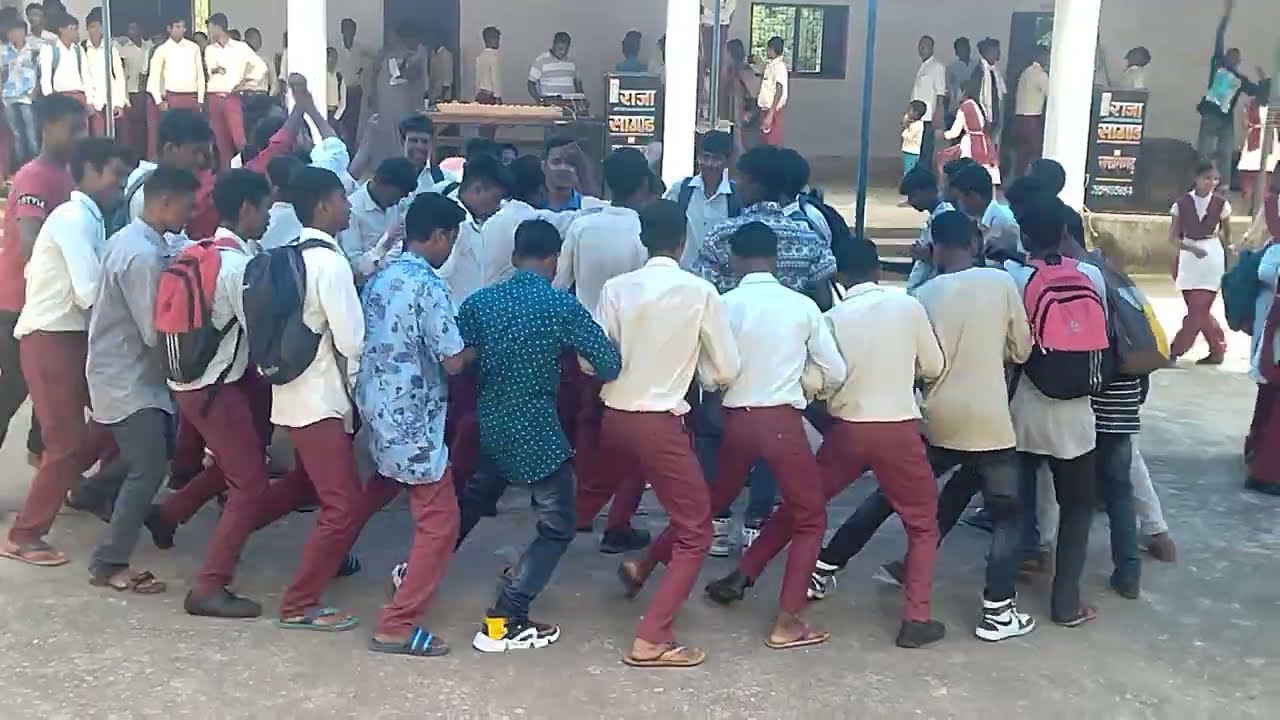The image depicts a large group, predominantly men with dark skin and black hair, likely of Indian or Asian descent, gathered outdoors in a central courtyard. They are positioned in a semicircle with their arms interlocked, appearing to engage in a unified dance or ritual. Many are dressed in maroon pants and white shirts, while others sport jeans and various colored clothing, including backpacks that hint at a younger crowd. The scene is set against a backdrop of buildings with people observing from a porch and other surrounding areas. The ground is paved, possibly asphalt or concrete, and the colors in the scene include gray, white, red, maroon, brown, blue, yellow, pink, and off-white. The atmosphere is lively, framed by the bright, sunny day.